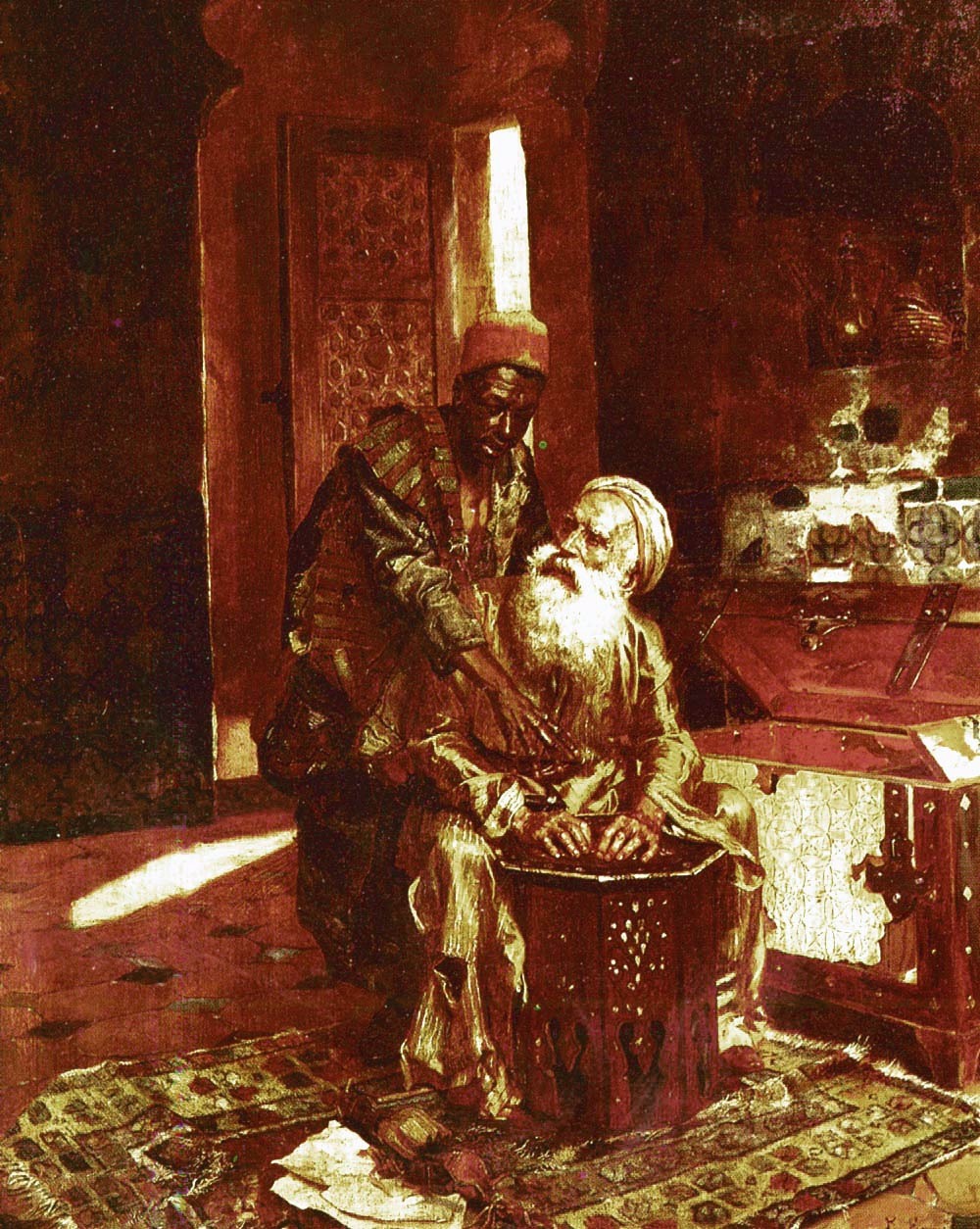The image is a detailed painting depicting an old, seated man with a long white beard and a gold turban. He is dressed in traditional flowing robes and sits with his legs wrapped around an octagon-shaped table, his hands resting on its surface. He gazes upward toward the side, where a black man stands behind him. This standing man is attired in traditional, old-fashioned clothing that features a brown and gold gown with matching pants, topped with a red felt hat and a shawl draped over his shoulders. The black man has one arm extended forward, pointing at something on the table.

Next to these two men, there is a large brown and gold chest, partially open, suggesting it holds several objects, possibly including a vase visible in the background. The setting appears to be an Arabic-style building, as indicated by the surrounding decor. The floor features a carpet with a gold diamond pattern, and the reddish flooring behind the table is similarly decorated. The walls are dark brown and gold, adorned possibly with images, creating a rich, historical ambiance. An open door behind the standing man allows sunlight to penetrate, illuminating the scene subtly and highlighting the intricate details. The entire setting, from the attire to the architecture, exudes an aura of antiquity, likely centuries old.